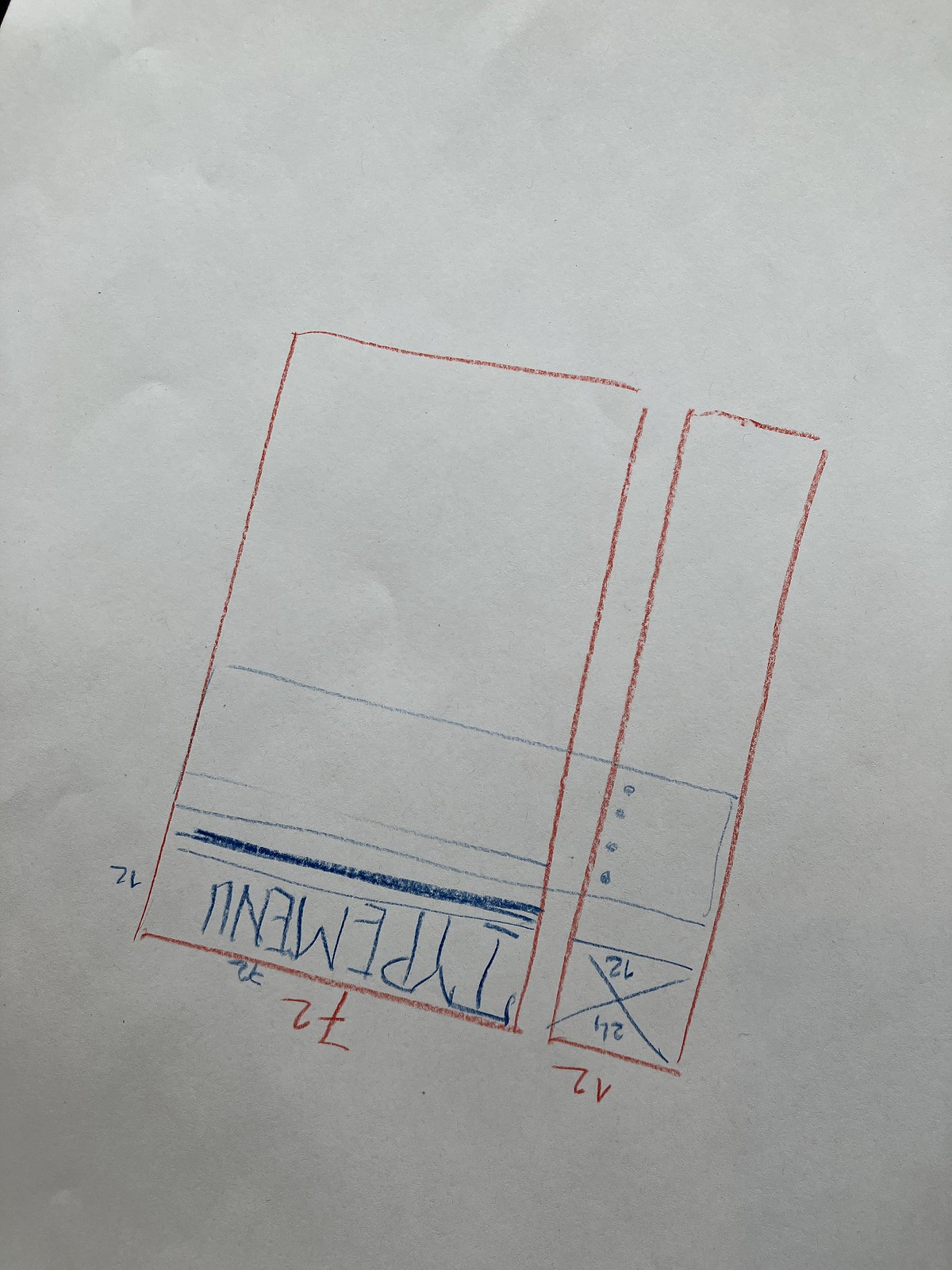In this detailed close-up photograph, a white sheet of paper takes up the entire frame, rendering itself the focal point with no other elements in view. The image is slightly grainy, emphasizing the texture of the paper. Tilted at a slight angle to the right, the photograph showcases a hand-drawn diagram comprising two adjacent red rectangles of identical height, seemingly sketched with colored pencils. The left rectangle is noticeably wider than the right one.

In the top half of the rectangles, there are no additional markings. Midway down, a blue horizontal line spans across both rectangles, followed by a series of four vertical dots aligned beneath it. Further down, another blue line traverses both rectangles. However, a subsequent horizontal line only appears within the left larger rectangle and does not extend into the right skinnier one. A thick blue vertical line is also present within the left rectangle.

Adding to the complexity of the drawing, there is some handwritten text, upside down, which reads "TYPE MENU", written messily but in all capital letters. Additionally, the numbers "7-2" appear twice, also upside down, and are written in blue pencil. The right rectangle features a red "X" with "26" adjacent to it and the number "172" written nearby.

Overall, the diagram is exclusively executed in red and blue colored pencil, with an assortment of lines, dots, and textual annotations creating an intricate and somewhat cryptic composition.